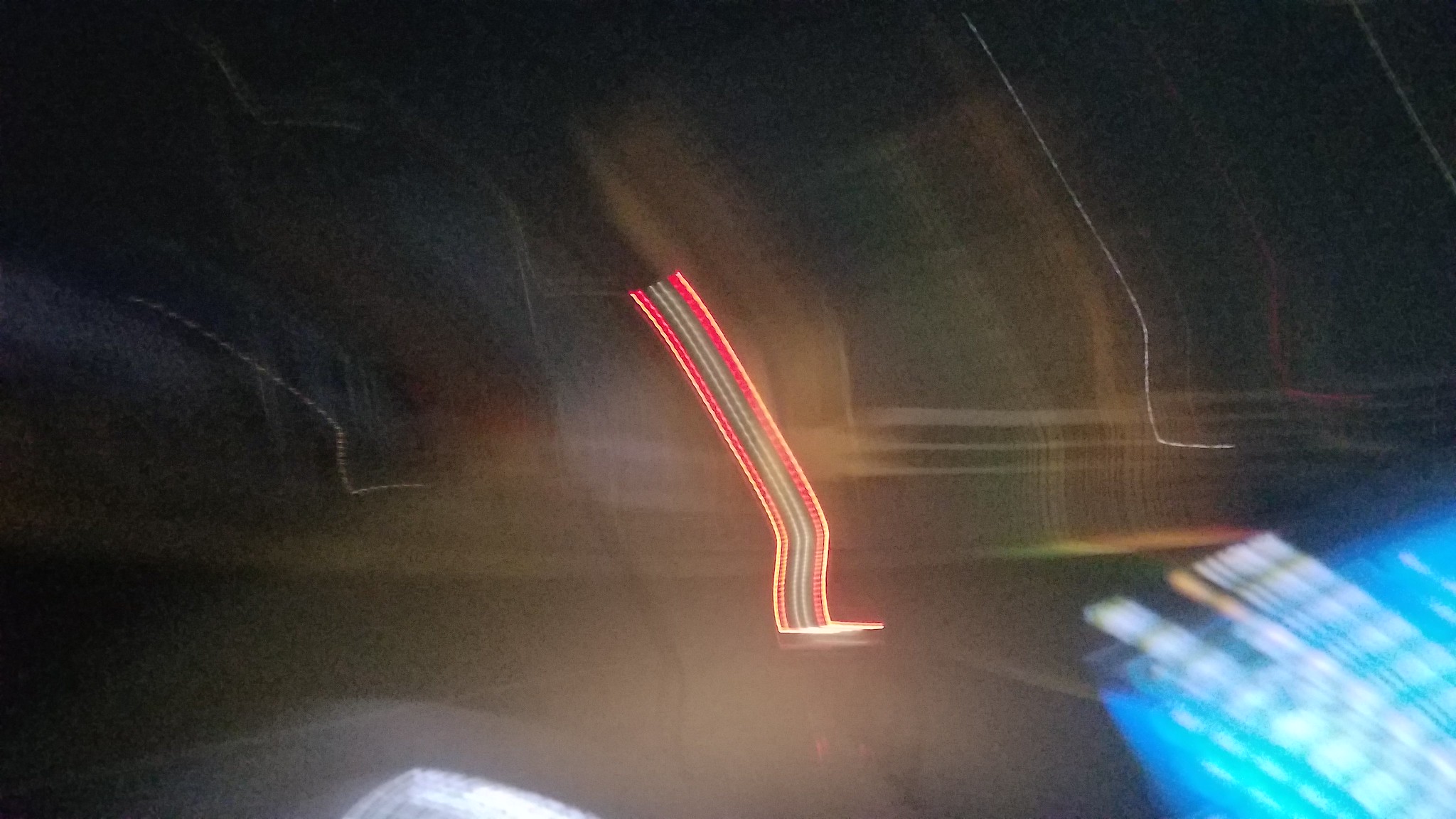A very blurry image features an intriguing array of lights. In the center, there are strips of neon lights arranged in a pattern that resembles a pants leg, complete with a distorted foot-like shape where the lights meet and bend on the floor. The pattern starts with a yellow band on one side, followed by red, black, gray, black, gray, red, and ends with another yellow band on the opposite side. The background is a psychedelic tapestry of colors, with numerous streaks flowing vertically from the top to the bottom of the image. In the bottom right corner, blue and white lights span upward from the edge, covering about a third of the image’s height.